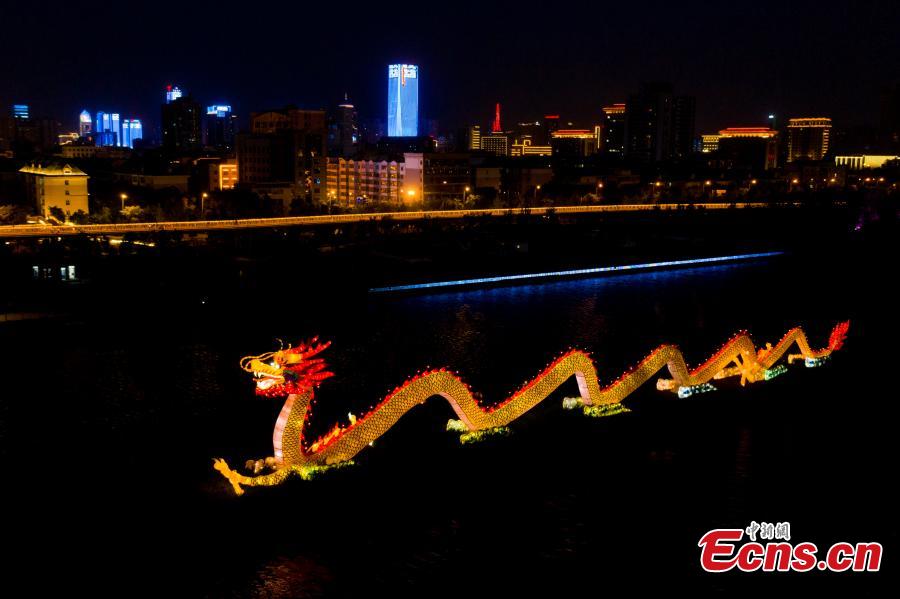The image is a vertical rectangular photograph captured at night, featuring a striking dragon sculpture floating on a pitch-black body of water. The dragon, colored in vivid shades of yellow and orange with a red-tinted head and facial features, weaves up and down along the water's surface. Its tail, decorated with a red feather-like element, adds to the impression of fire. The dragon's movement is aided by boats on either side, visible along the entire length of the sculpture. 

In the background, a city skyline with numerous buildings illuminated in blue, yellow, red, and gold hues is clearly seen. Streetlights dot the shoreline, and some homes with glowing white lights add warmth to the scenery. The reflections from the city's vibrant lights create streaks of blue and other colors on the water, amplifying the overall visual spectacle. 

Additionally, the lower right corner of the image contains a red logo with "ECNS.CN" in white text, accompanied by white-outlined Chinese characters above it.